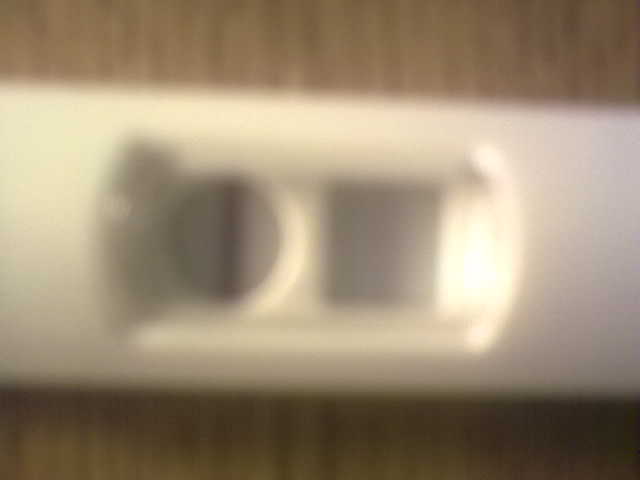This image captures an extremely close-up and blurry view of a white plastic pregnancy test resting on a light brown wood grain table. The focal point is the central section of the test, which features two small, indented windows: a circular one to the left and a square one to the right. A distinct pink line runs across the circle, indicating its test result, while the square window remains blank. Both windows are set into a rectangular depression with curved sides on the surface of the test. A bright light source reflects off parts of the rectangular depression, adding to the overall blurriness and making finer details difficult to discern.